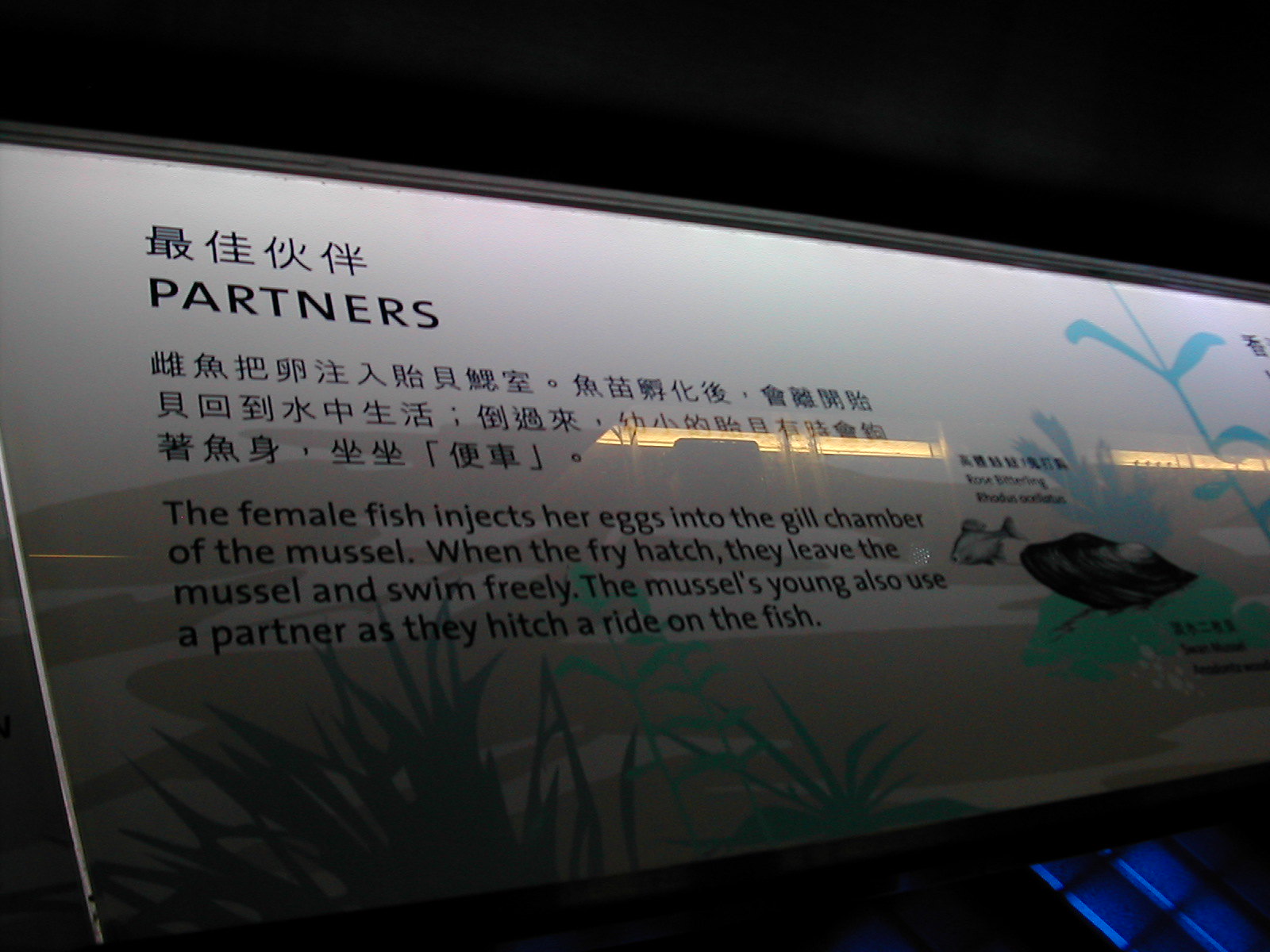This image depicts an informational sign, likely from an aquarium or wildlife area, featuring a glass or plastic screen in front of it. The sign is designed to educate viewers about aquatic life, specifically detailing the symbiotic relationship between a female fish and a mussel. The text on the sign is presented in both English and an Asian language, most probably Japanese.

At the top left corner, the sign features the heading "Partners" in English, followed by a paragraph of explanatory text. It reads: "The female fish injects her eggs into the gill chamber of the mussel. When the fry hatch, they leave the mussel and swim freely. The mussel's young also use a partner as they hitch a ride on the fish." This English text is mirrored by a corresponding translation in Japanese below it.

To add a visual element, the sign includes a painting of an underwater habitat complete with fish and various aquatic plants, adding context to the information provided. On the right side of the sign, there are illustrations of two fish species, each labeled with their common and scientific names. One of the species mentioned is the rose bitterling. The background of the sign is predominantly white with green and blue vegetation accents, creating an engaging and informative display.